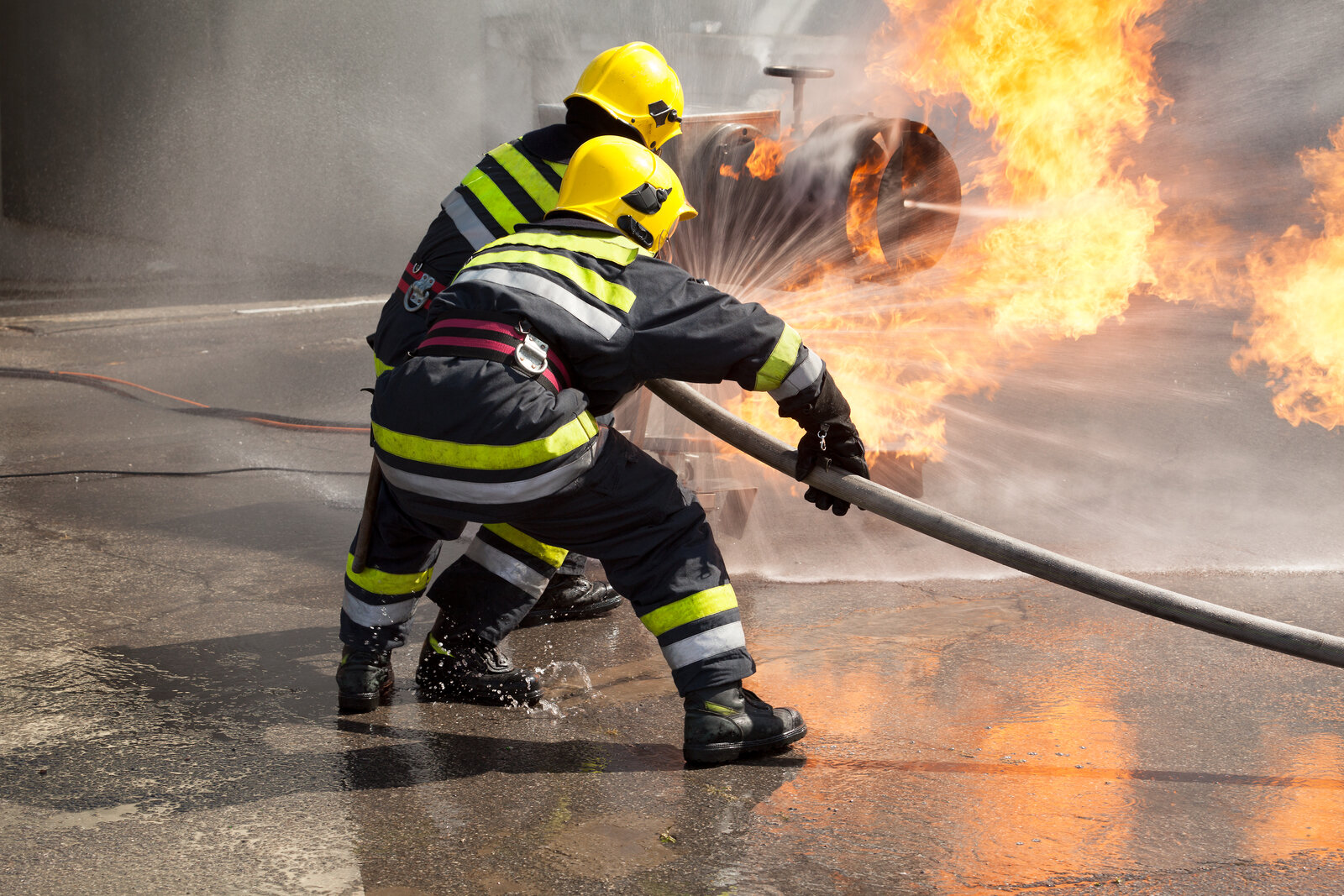This image captures a live-action moment of two firefighters engaged in a controlled demonstration, battling a large flame erupting from a pipe. The scene is set on a wet asphalt surface, likely a driveway or parking lot, with smoke billowing in the background. Both firefighters are wearing full protective gear, including black fire-retardant suits adorned with fluorescent yellow and silver reflective stripes, yellow helmets, black gloves, and boots. The firefighter at the back steadies the gray hose, while the one in front operates the water blaster, producing a dome of water that covers the fire. The ground beneath them is completely saturated, highlighting the intensity of their efforts.